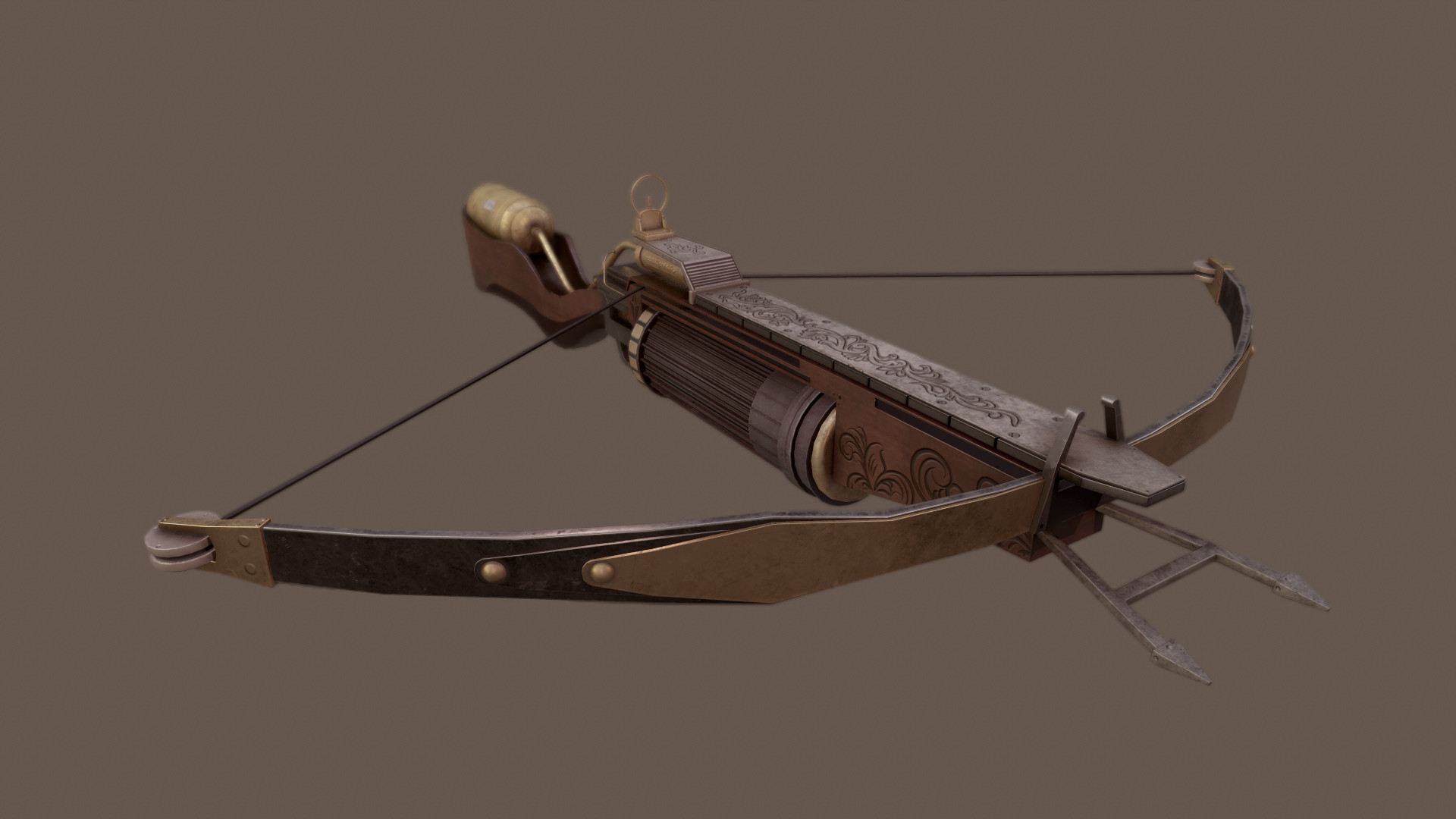The image showcases a detailed, intricately designed crossbow rendered against a neutral grey background, which suggests it might be an asset for a video game or a conceptual design. The crossbow is depicted from a front-side angle, with its body extending diagonally from the top left to the bottom right of the image. The bow runs horizontally with pulleys at the ends, although it doesn't appear to be a compound bow, as the visible string is only the one that would propel the bolt. The crossbow is not loaded, but its sights are positioned at a bronze collar. 

The stock, which appears to be made of light wood featuring a pocket that might hold small items, doubles as a crank and is adorned with an iron piece that has a swirly, regal design. The round hand grip is located in front of the taut bowstring. Notably, two sharp, fixed prongs extend from the front end of the crossbow, resembling bayonet analogs for close combat situations. There are no figures, text, or additional drawings in the image, focusing all attention on the detailed and functional aspects of the crossbow.